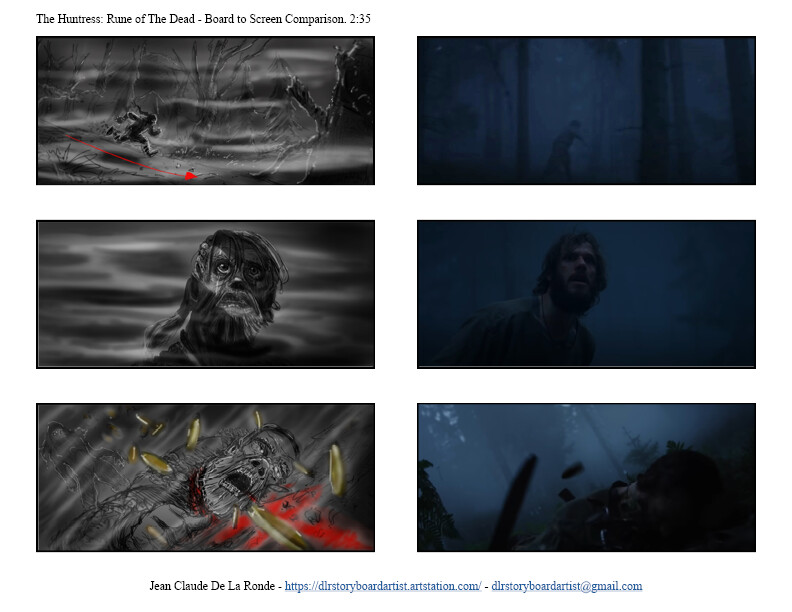This image is a collage of six horizontal rectangles arranged in three rows and two columns, serving as a storyboard-to-screen comparison for a movie. At the top, the text reads: "The Huntress: Rune of the Dead - Board to Screen Comparison 2.35." The left column contains black and white storyboard sketches, while the right column features their corresponding live-action movie scenes in darker tones of blue and black. 

- In the first row, the storyboard shows a person running through the woods, with the adjacent movie clip capturing the same frantic motion.
- The second row depicts a bearded man's head emerging from the mist in the storyboard, mirrored by the live-action shot of the actor in the mist.
- The third row illustrates a dramatic scene where an individual lies amidst flying bullets in the storyboard, matched by the live-action shot showing the man on the ground with bullets surrounding him.

At the bottom, the text states: "Jean-Claude De La Ronde - https://DLRstoryboardartist.artstation.com - DLRstoryboardartist@gmail.com." 

This detailed comparison highlights the translation of initial concepts into final film sequences.